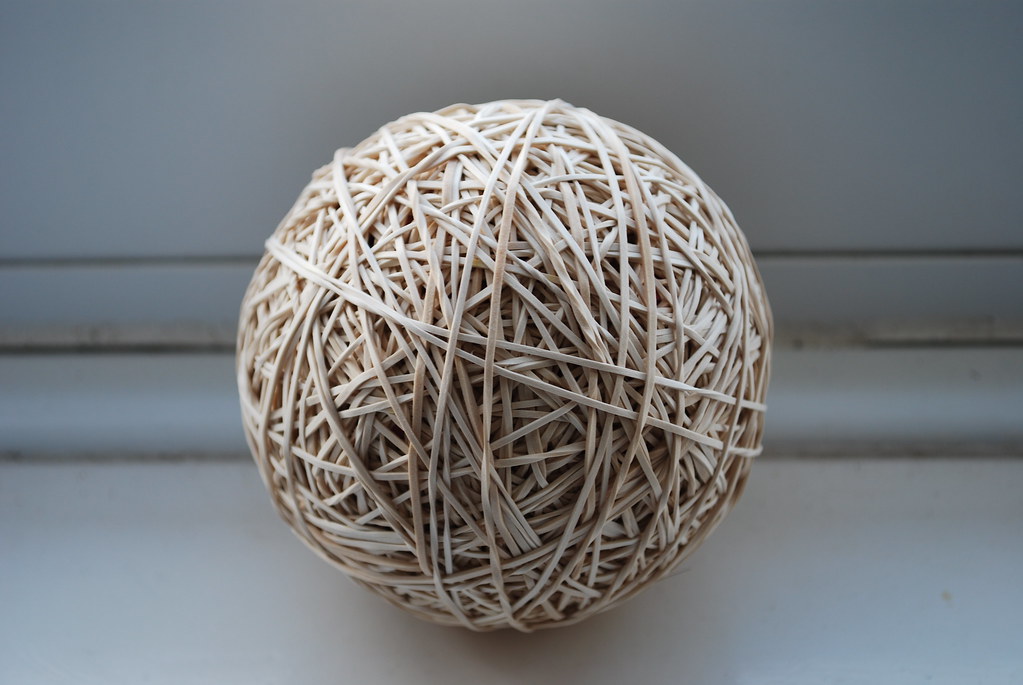The image features a large, meticulously crafted rubber band ball, composed of countless white to beige rubber bands intricately wrapped around each other to form a perfectly round sphere. The ball is prominently placed at the center of the photograph, dominating the frame. A bright light from the top-left corner illuminates the upper portion of the ball, casting detailed shadows that highlight the individual bands, with darker tones visible underneath. The background consists of a gray, slightly blurry floor and a similarly colored wall, creating a neutral backdrop that accentuates the ball. This visually striking piece could be either an actual rubber band ball or an artfully designed sculpture mimicking one, celebrated for its detailed construction and placement.